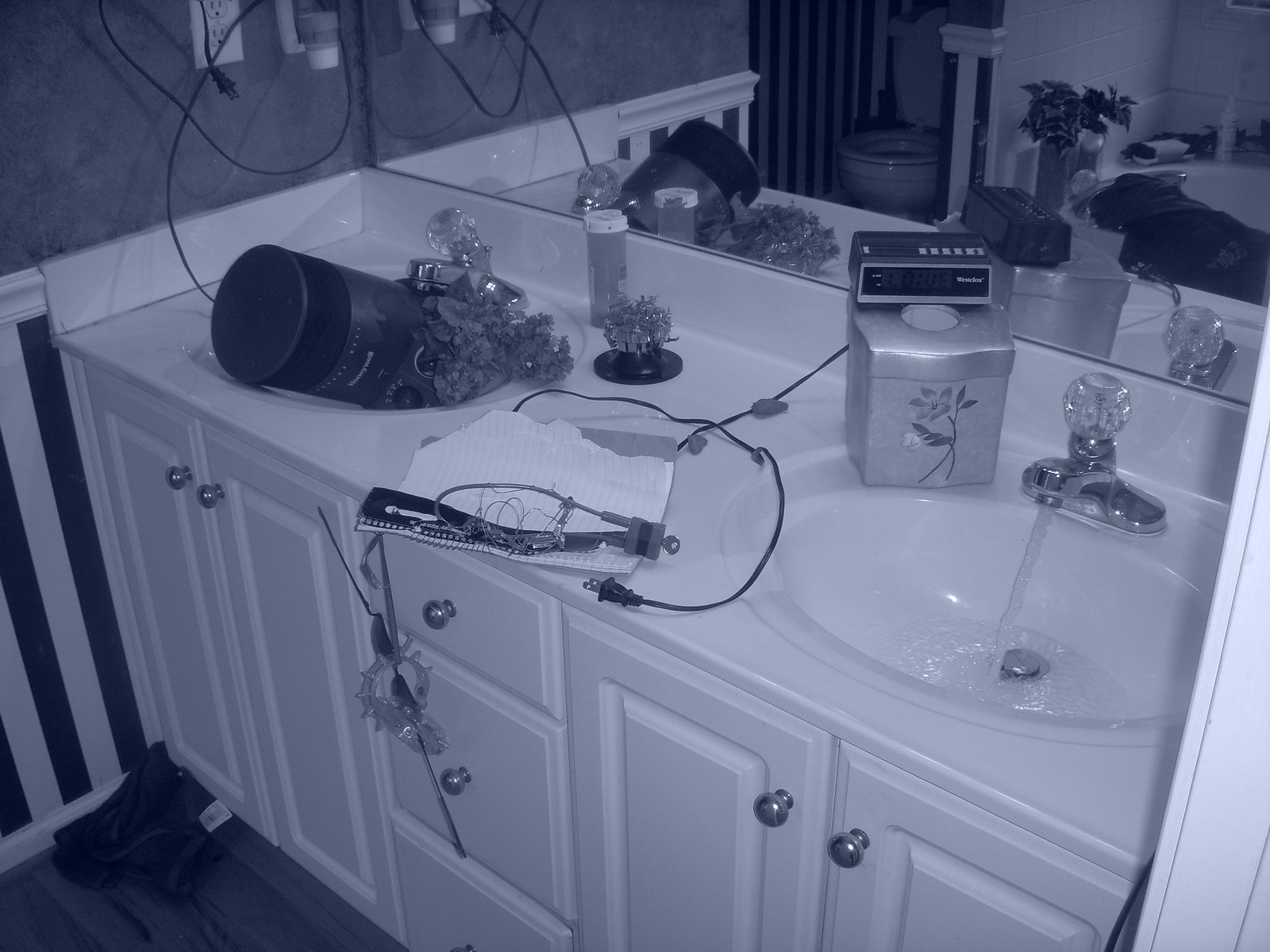This black and white photograph captures a cluttered bathroom scene featuring two sinks. The left sink is occupied by a pair of fake flowers, a large bottle of medication, and a small space heater with its plug wrapped around a wall-mounted Dixie cup holder. The counter between the sinks is strewn with papers and miscellaneous trash. Adjacent to the right sink, a container of wipes sits with an unplugged alarm clock perched on top, its cord tangled among the papers. The water in this sink is running, though the open drain prevents it from pooling. Reflected in the mirror, the background reveals a bathtub accompanied by a white porcelain toilet. Nearby, more fake plants add to the decor. The bathtub's edge is cluttered with assorted bath products and what appears to be a robe. The overall image evokes a sense of disarray within the bathroom.